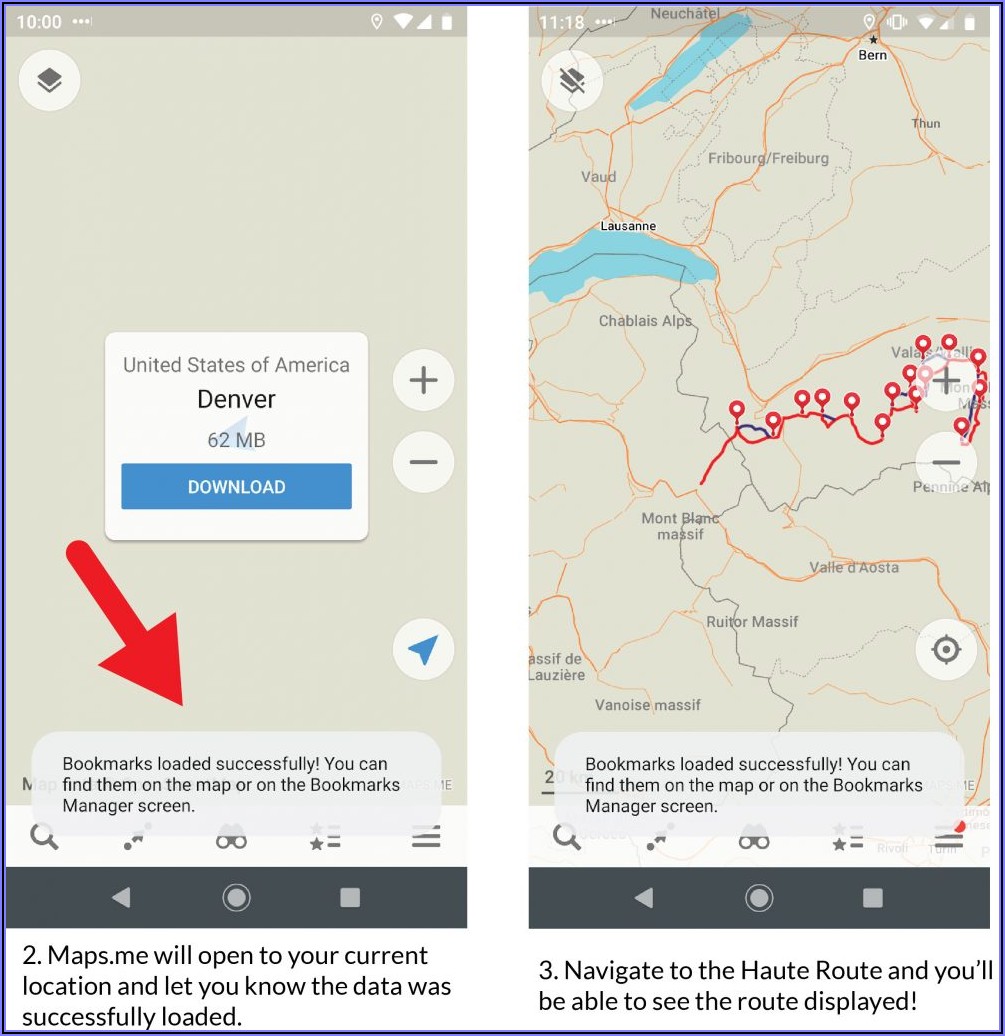The image is a vertical rectangle framed by a purple-blue border. It contains two adjacent cell phone screenshots. The left screenshot shows a device interface indicating the time as 10 o'clock, with an array of symbols at the top: three horizontal dots on the left and icons for location, Wi-Fi, cellular signal, and battery on the right, all displayed within a brownish-gray bar with white text.

Below this bar, there's a beige background featuring a pop-up window with the following details: "United States of America, Denver, 62 megabytes" and a blue "download" button with white text. Adjacent to the pop-up, plus and minus symbols are visible.

Additionally, a large red arrow points diagonally downwards to a caption that reads, "Bookmarks loaded successfully. You can find them on the map or on the bookmarks manager screen." Below this notification is a black border containing icons for a back arrow, a circle, and a square. At the very bottom, text states, "maps.me will open to your current location and let you know the data was successfully loaded."